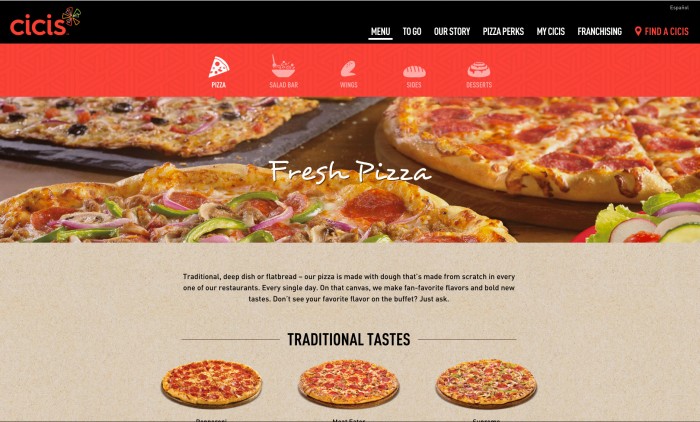This detailed screenshot from CeCe's Pizza website showcases their various menu options. The top section of the image features a black rectangular banner with the text "CeCe's" prominently displayed, extending across the width of the screen. Below the banner, a navigation menu includes options such as "Menu To Go," "Our Story," "Pizza Perks," "My CeCe's," "Franchising," and "Find a CeCe's," with the "Find a CeCe's" option highlighted in red.

The main background is a vibrant red, listing categories such as "Pizza," "Salad Bar," "Wings," "Sides," and "Desserts." The "Pizza" and "Menu" buttons are selected, revealing an array of pizza options. The selection includes "Flatbread," "Traditional Deep Dish," and "Thin and Crispy" varieties.

An informative section emphasizes that CeCe's pizzas are crafted with dough made fresh from scratch in every restaurant, every day. This fresh dough serves as the base for a variety of popular flavors and innovative new options. The text also invites customers to request their favorite flavors if they are not available on the buffet.